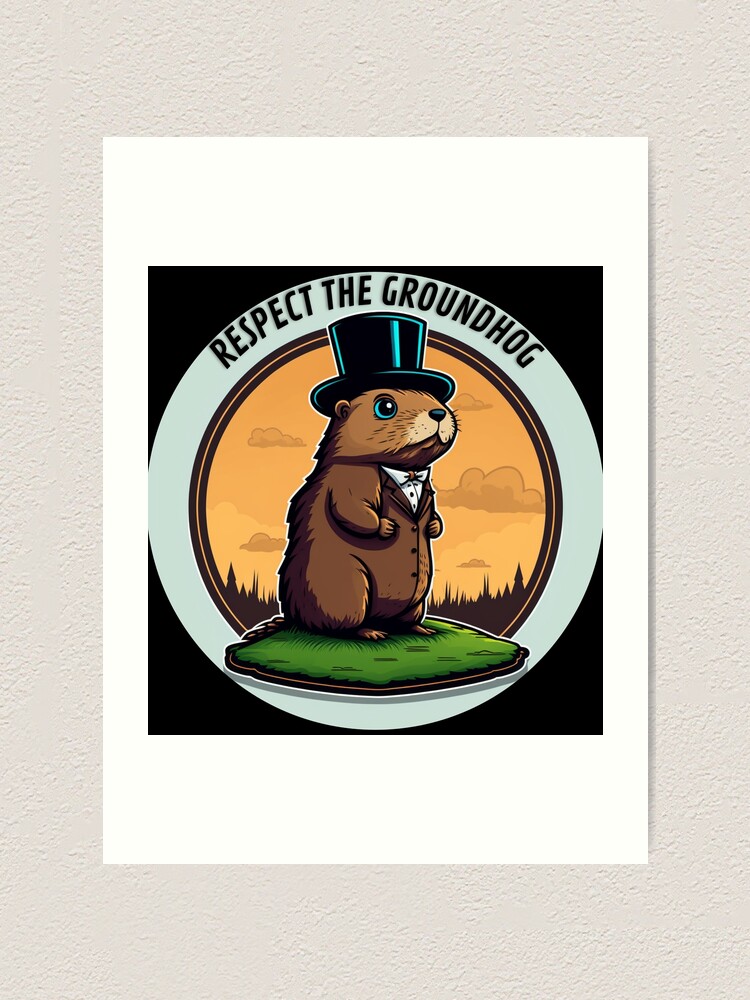The image features a detailed illustration of a groundhog standing upright against a white circular backdrop. This white circle sits at the center of a layer of black paper, which is itself placed against a beige background. The thick white circle prominently displays the phrase "RESPECT THE GROUNDHOG" at the top in large, bold black letters.

In the forefront of the image, the groundhog is depicted in intricate detail. It sports a classic top hat and a brown suit coat, paired with a white shirt and a matching white bow tie. The groundhog is oriented towards the left, gazing off into the distance with expressive brown eyes that have black centers. Its muzzle is lighter in color, and it has a distinctive black nose. The groundhog’s hands rest gently against its chest, aligning with its coat.

Surrounding the groundhog at the base of the circular background is a green patch of grass that adds a natural element to the scene. The sky behind the groundhog is painted a warm orange, suggesting either dawn or dusk. Adding to the depth of the setting, black silhouette trees with pointed tops can be seen in the distant background, further enriching the overall composition of the artwork.